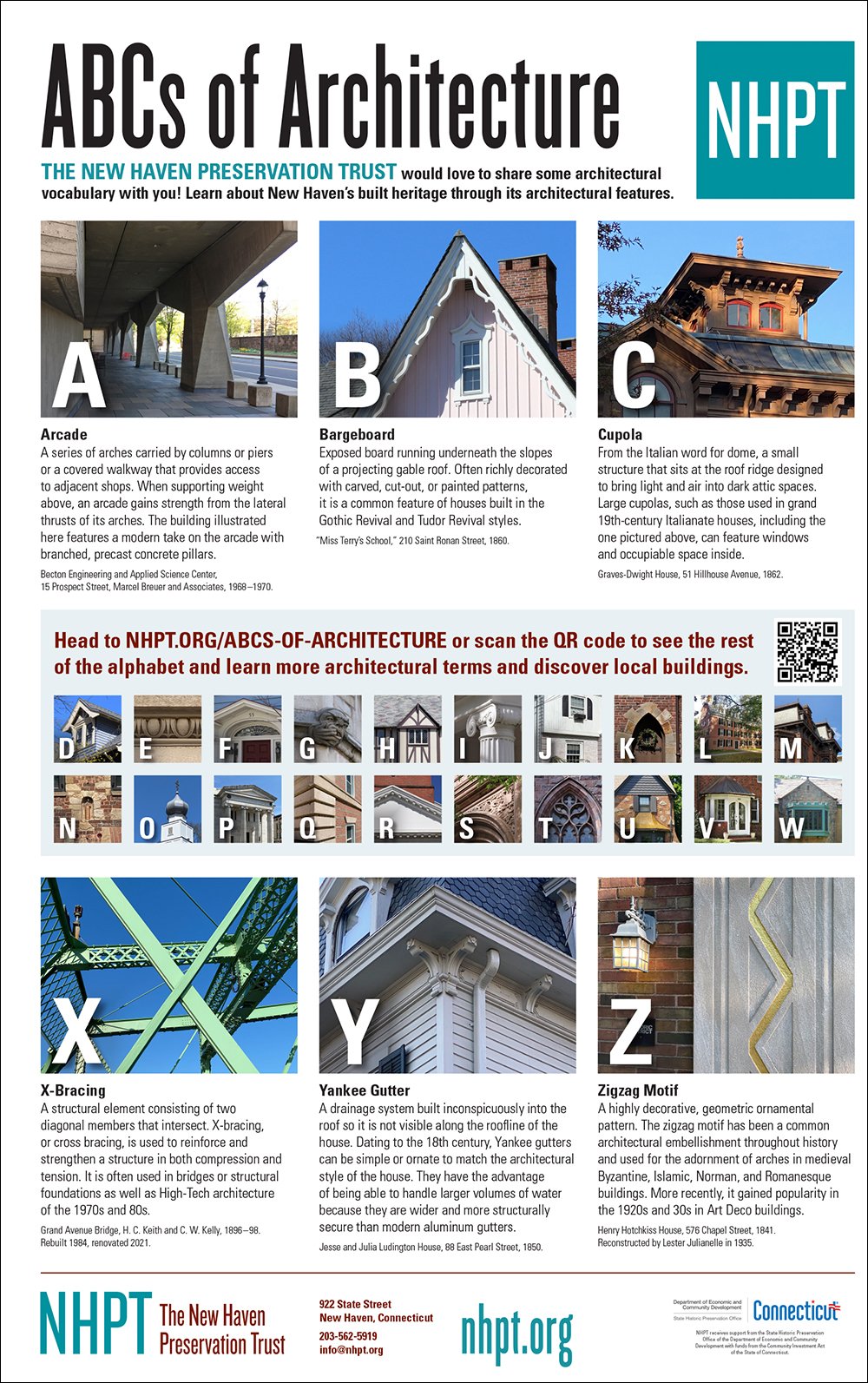The image is a horizontally oriented page, likely from a magazine or a book, detailing various architectural terms. At the top, in large black letters, it states "ABCs of Architecture." Below this title, a blue rectangle on the right contains the white letters "NHPT," representing the New Haven Preservation Trust. The accompanying text reads, "The New Haven Preservation Trust would love to share some architectural vocabulary with you. Learn about New Haven's built heritage through its architectural features."

The layout features the letters A through Z, with the letters A, B, C, X, Y, and Z prominently displayed in larger images. The images corresponding to A, B, C showcase architectural elements: "arcade" under A, "bargeboard" under B, and "cupola" under C. Each image is accompanied by a paragraph explaining its term. 

In the middle section of the page, smaller images representing letters D through W display various architectural features of houses and buildings, each with its descriptive text. At the very bottom, the page highlights "X bracing," "Yankee gutter," and "zigzag motif" with larger images, continuing the theme of architectural education.

The image also includes the NHPT website information, NHPT.org, reinforcing its educational intent about New Haven's architectural heritage.